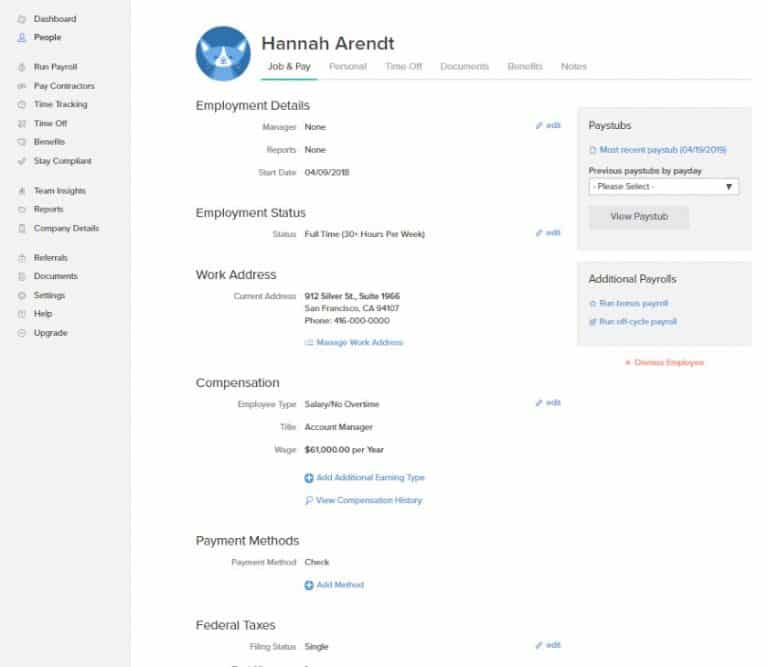This image displays a detailed profile screen for an employee named Hanna Arendt, spelled H-A-N-N-A-H A-R-E-N-D-T. At the top of the screen, Hanna's name is prominently displayed, followed by sections labeled "Job and Pay," "Personal," "Time Off," "Documents," "Benefits," and "Notes," with a green underline emphasizing the active "Job and Pay" section. To the left of Hanna's name, a teal and deep blue cartoon-like cat serves as her profile picture.

The screen under "Job and Pay" features an "Employment Details" section, indicating no manager or direct reports. Hanna's employment start date is listed as April 9, 2018. Further down, her employment status is marked as "Full Time," with a specification of working 30-plus hours per week. Her work address is provided, showing her current location in San Francisco, California.

Additional details include a phone number for contact and a section to message her work address. The profile also contains dedicated areas for viewing pay stubs, additional payrolls, compensation details, and payment methods, specifying that Hanna receives her payment via check. Federal taxes information is also available. At the bottom right corner of the screen, there is a small edit button for making updates to her profile.